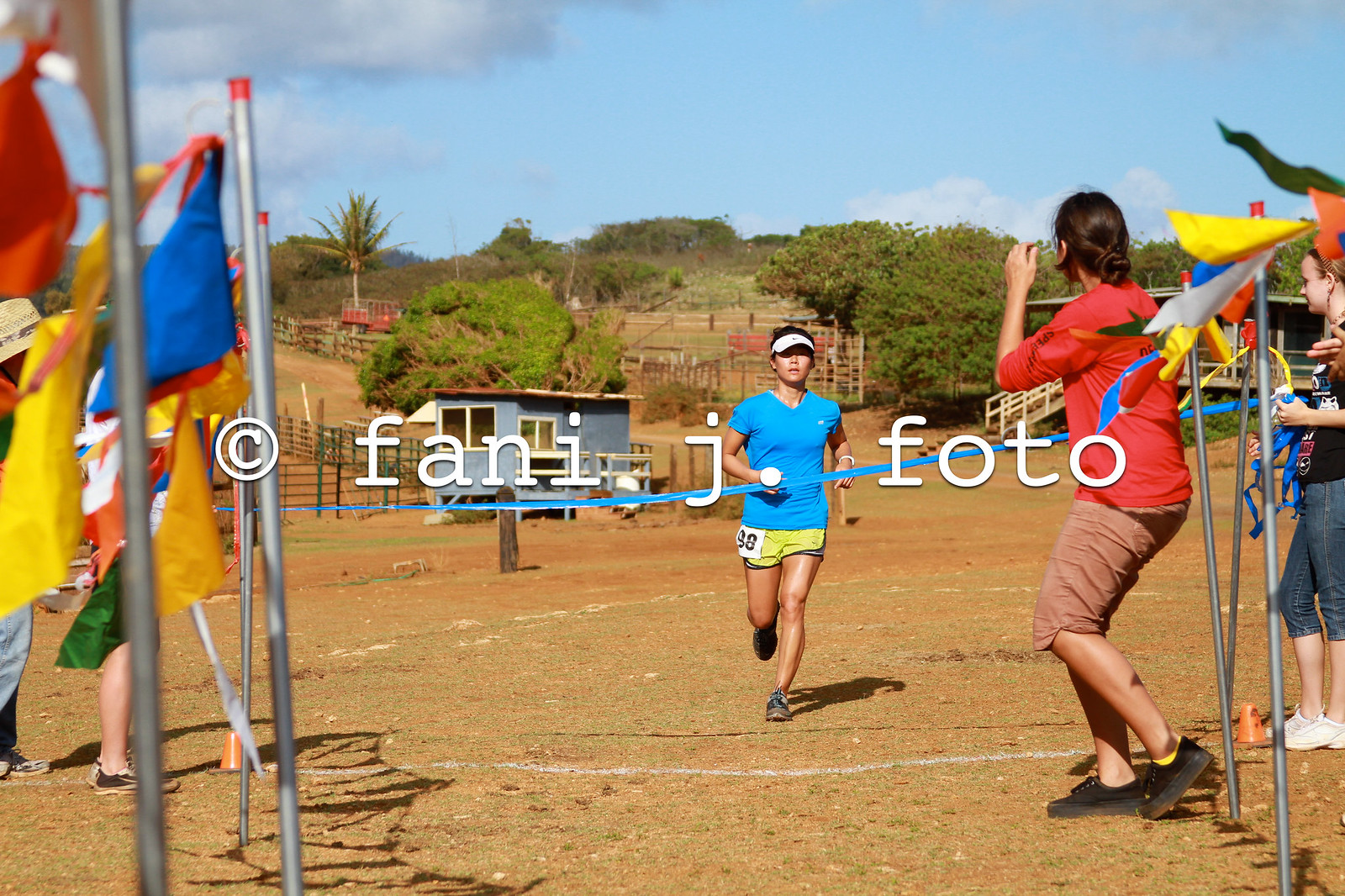In this photograph, a female runner is captured mid-stride as she approaches the finish line of what appears to be an outdoor rural marathon, possibly held in an Asian country. She's wearing a turquoise v-neck top, lime green shorts with a white tag numbered 98, and a white visor. The setting features a symbolic finish line marked by a ribbon held by a girl on one side, with colorful flags—blue, red, yellow, green—lining the path on both sides, fluttering from metal poles.

The runner's path is delineated by a white chalk line drawn across the tan, brown dirt, indicative of the warm, farmland environment, further emphasized by the presence of a small blue hut and a palm tree in the background. The ground is a mix of dead grass and brown dirt. A copyright overlay in white font reading "fanny.foto" is visible at the center of the image.

Several onlookers are gathered near the finish line, cheering her on. Notably, a man in a red shirt, brown pants, and black sneakers, with long hair tied back in a bun, is enthusiastically clapping with his arms raised. The vibrant scene captures the communal spirit and the enthusiasm of the spectators as they eagerly await the runner’s completion of the race.